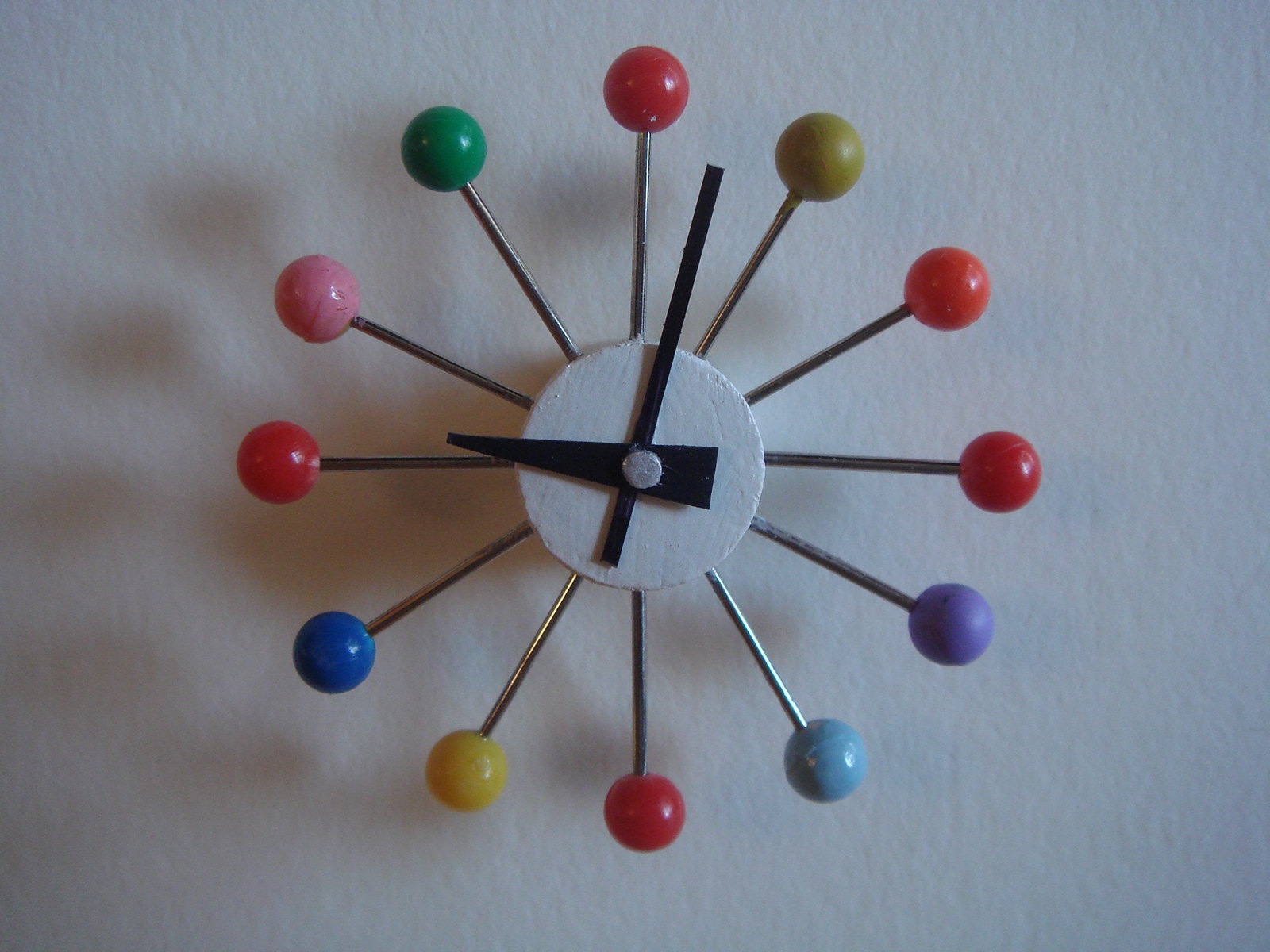The image features a distinctive clock mounted on a white wall. The clock's design departs from traditional numbers, using 12 steel rods, each ending in a colorful ball, to mark the hours. The balls vary in color, including red at the 12, 3, 6, and 9 o'clock positions, green at 1 and 11 o'clock, orange at 2 o'clock, purple at 4 o'clock, blue at 5 and 8 o'clock, yellow at 7 o'clock, and pink at 10 o'clock. The black hour and minute hands point to 9:03. A small white circle forms the center of the clock, and the entire piece casts a shadow on the wall behind it.